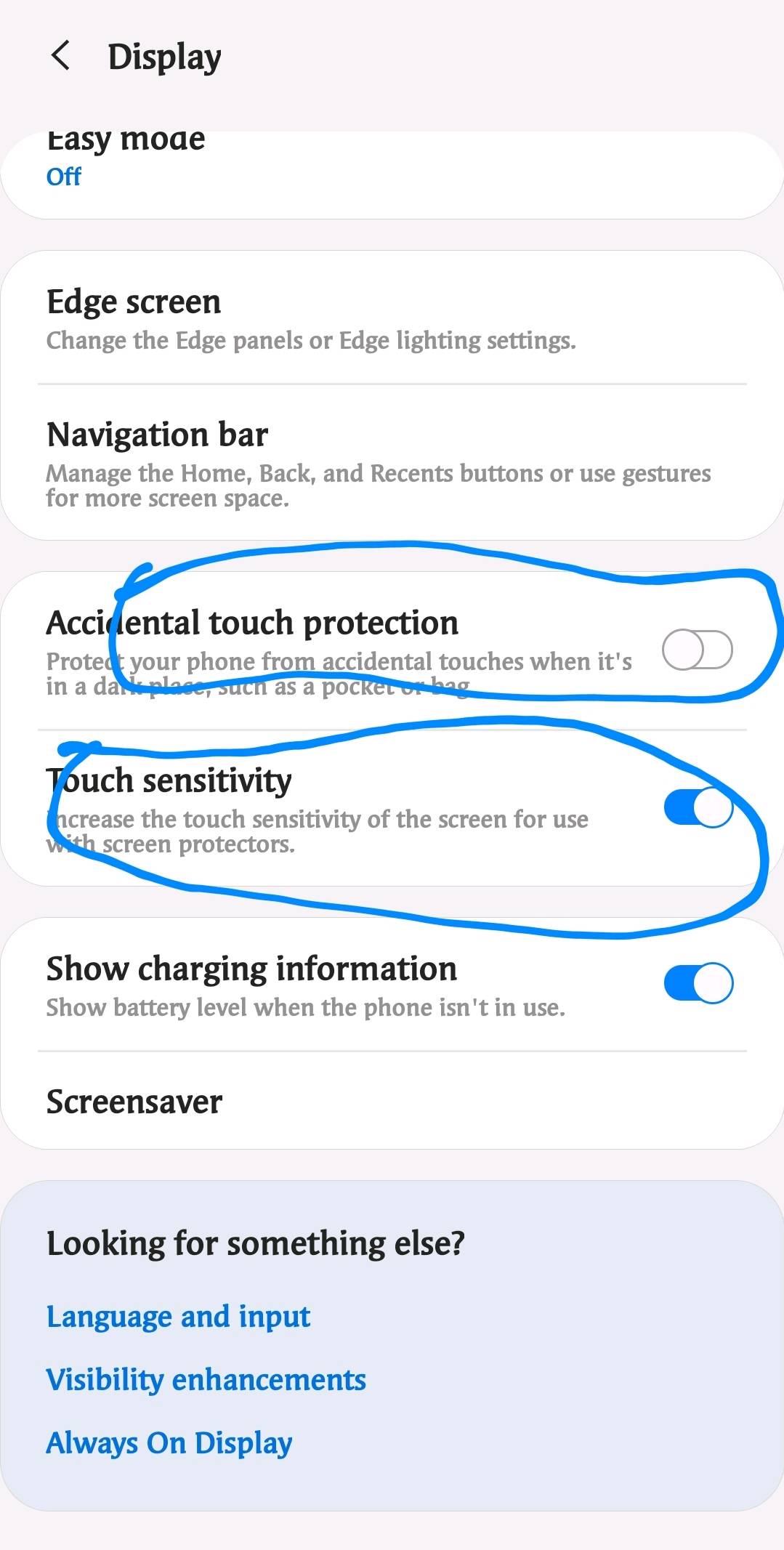The image displays a smartphone settings menu with various options, organized under different sections. At the top, the "Display" settings category is prominently visible. Below that, the first option titled "Easy mode" is shown as turned off. 

Under the "Easy mode" section, there is a bold heading, "Edge screen." The next line, in regular text, reads "Change the edge panels or Edge lighting settings."

Next, a boldly labeled section, "Navigation bar," is followed by an explanatory line in regular text: "Manage the Home, Back, and Recent buttons or use gestures for more screen space."

Beneath this, a section titled "Accidental touch protection" includes a description: "Protect your phone from accidental touches when it's in a dark place such as a pocket or bag." This option has a toggle bar positioned to the left, indicating that it is turned off, and the entire section is highlighted with a blue circle.

Further down, the "Touch sensitivity" option comes with the description: "Increase the touch sensitivity of the screen for use with screen protectors." Here, the toggle bar is turned to the right and shown in blue, signifying that it is enabled, and the section is also circled in blue.

At the bottom of the menu, the entry "Show charging information" reads: "Show battery level when the phone is in use," indicating its purpose.